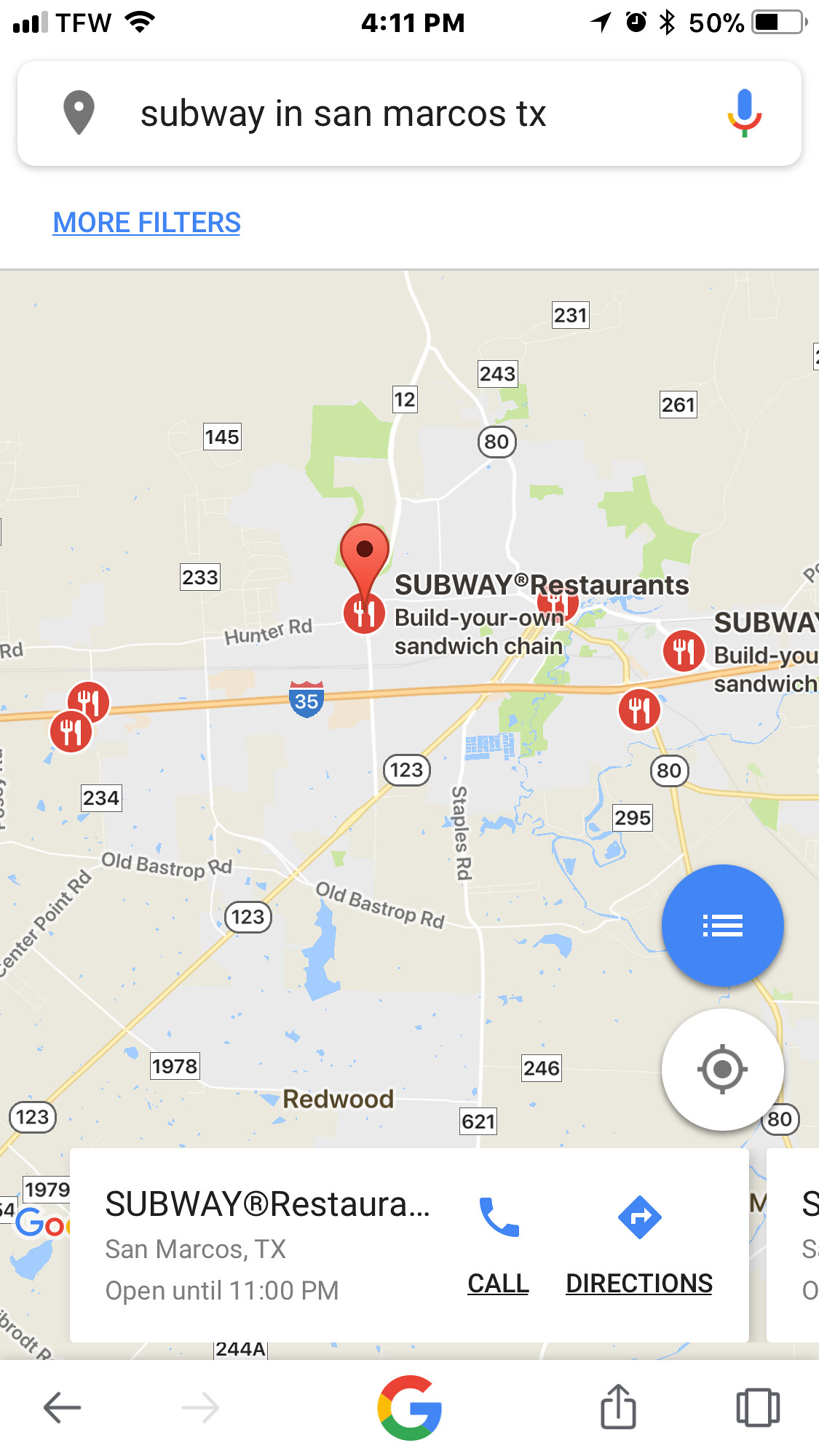This is a screenshot from a smartphone depicting a search for Subway restaurant locations in San Marcos, Texas. At the top of the screen, the search bar confirms the query, "Subway in San Marcos, Texas." Below it, a map of the San Marcos area is visible with multiple Subway locations marked by pins. Notably, there are two Subway pins on the far left side along Interstate 35, positioned towards the center of the map as it runs horizontally. Similarly, there are two other Subway pins on the right side of Interstate 35, also aligned horizontally. The most prominent pin, appearing larger than the others, is located in the upper third of the screen, just north of Interstate 35. At the bottom of the screen, there are options to either call the Subway restaurant or get directions to it.